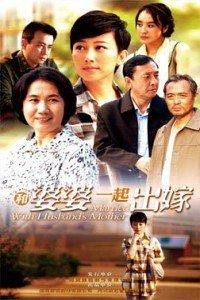This detailed movie poster, possibly an advertisement originating from China or Central Asia, is divided into two distinct halves with text, likely in Chinese, positioned between them. The upper half showcases a diverse group of characters, all appearing to be Asian and suggesting a familial bond or perhaps representing different important figures in the storyline. Among them is a younger girl wearing a plaid shirt, an elderly woman with gray hair, a man dressed in a business suit with a blue shirt, and other individuals with varying appearances and ages.

The lower half of the poster features the young girl from the top section, now seen with her fist raised thoughtfully to her chin as she walks across a crosswalk. This part of the image is imbued with a yellow-orange tint, enhancing its visual appeal. The two sections are separated by a white blurred border, adding to the artistic composition of the poster. The overall design and character presentation strongly suggest that this is a promotional piece for a dramatic or familial-themed movie.